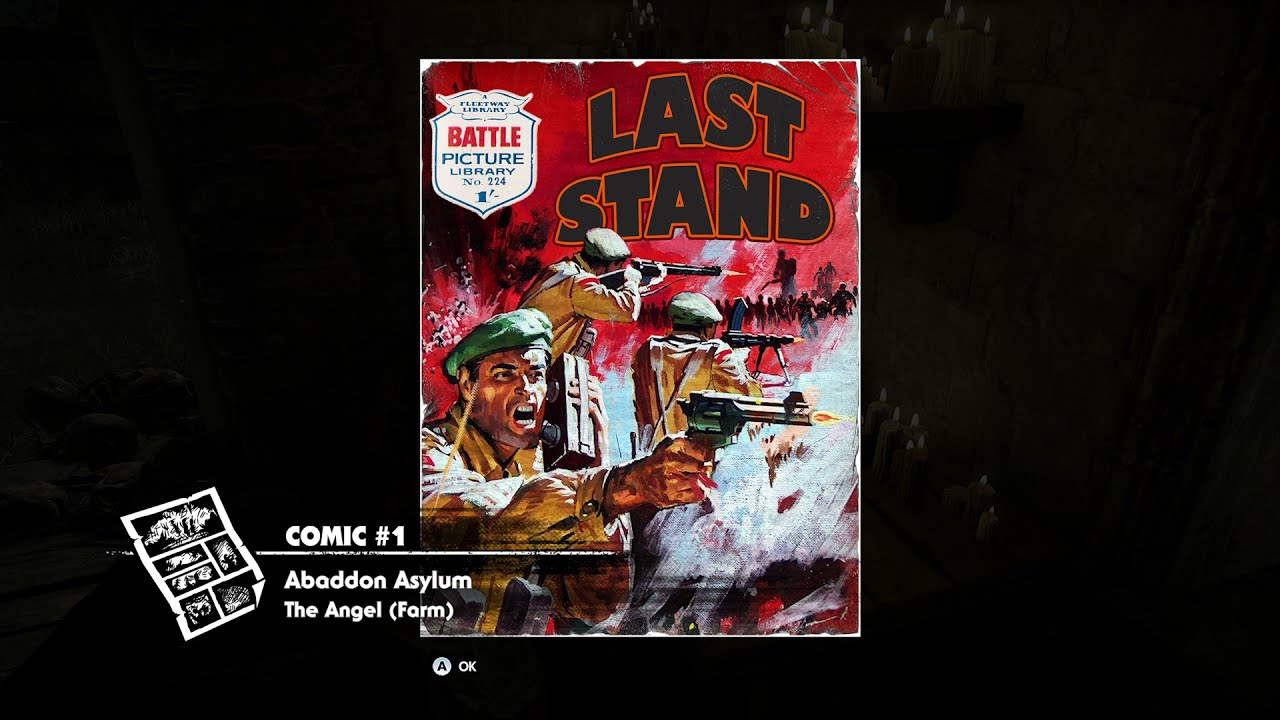The image depicts a highly detailed and graphic comic book cover titled "Last Stand." Dominating the scene is a chaotic war setting with numerous soldiers, each embroiled in intense firing. The central figure, a soldier with a gun in his right hand from which flames are erupting, stands out prominently against the backdrop of a vivid red sky. Other soldiers are positioned behind him, their backs turned as they aim and shoot in various directions. In the upper left corner of the cover, a distinctive shield-like icon reads "Battle Picture Library" with "No. 224" subtly below it. Additionally, at the bottom, there is a small "A for OK" logo, suggesting that this comic might be accessible online. The image's thumbnail appears folded at the upper right corner and features a notable white circle on a blue background on the upper left, while the lower left and right corners display green and a white diagonal bar, respectively.